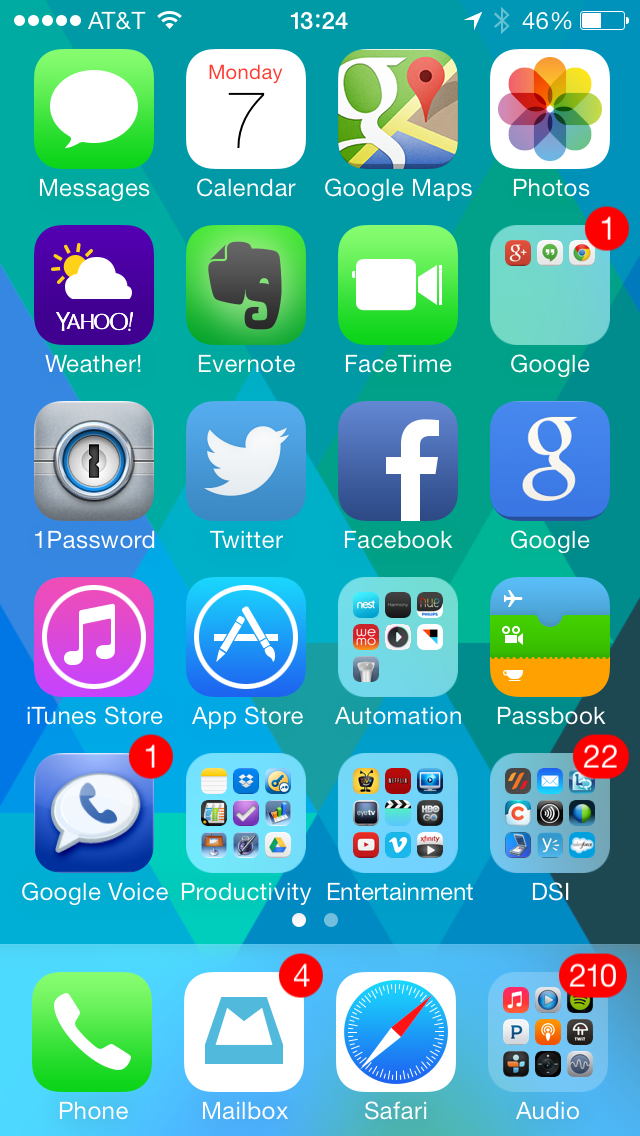This image showcases the home screen of a smartphone, meticulously detailing the layout of the apps and interface elements. Starting from the top left corner, there are five signal strength circles adjacent to the text "AT&T" in white. To their right, a fully filled Wi-Fi symbol is visible. Centrally positioned at the top is the time, displayed as "13:24". Moving to the top right corner, the battery icon is half-filled, accompanied by "46%" indicating the battery charge left.

Just below this status bar, several rows of app icons are arranged in a grid. 

- **First Row (left to right):**
  - **Messages:** Represented by a green speech bubble icon.
  - **Calendar:** Displays "Monday" and the number "7" on the icon.
  - **Google Maps:** Features a large "G" symbol.
  - **Photos:** Icon typically represented by a colorful flower.

- **Second Row:**
  - **Weather:** Usually depicted with a sun or cloud icon.
  - **Evernote:** An icon with an elephant logo.
  - **FaceTime:** A green camera symbol.
  - **Google:** Likely showcasing the "G" logo again.

- **Third Row:**
  - **1Password:** An app known for its vault icon.
  - **Twitter:** Recognized by the blue bird icon.
  - **Facebook:** Depicted with the iconic white "f" on a blue background.
  - **Google (duplicate):** Another instance of the Google "G" logo.

- **Fourth Row:**
  - **iTunes Store:** Represented by a star in a purple circle.
  - **App Store:** The blue icon with an "A".
  - **Automation:** Likely featuring a settings gear or similar icon.
  - **Passbook:** Typically shown with a stack of cards.

- **Fifth Row:**
  - **Google Voice:** Known for its phone and chat bubble icon.
  - **Productivity:** Represented by a relevant icon symbolizing productivity tools.
  - **Entertainment:** Likely featuring a play button or a related symbol.
  - **DSI:** An app with a specific icon not detailed here.

- **Bottom Dock (left to right):**
  - **Phone:** Green icon with a phone receiver.
  - **Mailbox:** Blue icon resembling an envelope.
  - **Safari:** Compass icon.
  - **Audio:** Typically represented by music notes or sound waves.

The background of the home screen is a gradient of greenish-blue hues, contributing to a serene and calming visual aesthetic.